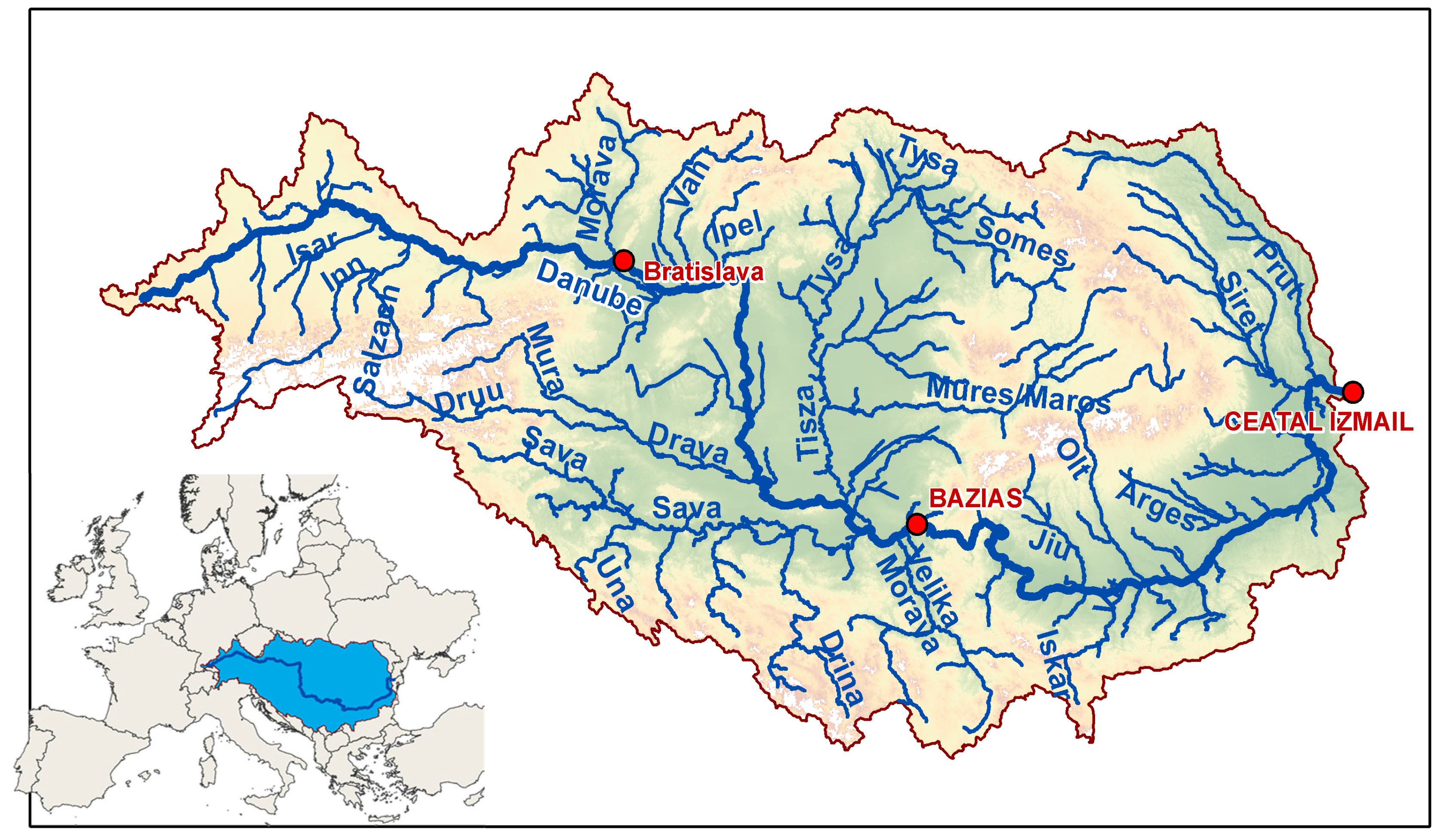This detailed image showcases a historical topographical map bordered in black, featuring two inset images for context. The inset on the left provides a larger global view, highlighting a land mass, bright blue against a grayish world background. This same land mass is then isolated and vividly colored in shades of yellow, green, and red on the main map, suggesting elevation and topography. 

The primary map depicts a region to the east of France and Italy, focusing extensively on its river systems. Key rivers such as the Danube, Sava, Tisa, and Prut are prominently labeled, along with numerous smaller tributaries including Izir, Salza, Murra, Danub, Morev, Va, Dreya, Seya, Una, Drina, Moreva, Tiza, Soms, Mores, Moravs, Arges, Olt, Ju, Iskar, Siret, and Sire. The waterways are illustrated in dark blue, contrasting against the pale yellow and green hues of the map, which may indicate varying terrains.

Additionally, the map features three notable red dots marking important locations: Bratislava in the upper left, Basias centrally, and Sieta Izmal (also referenced as Getal Ismail) on the far right. The intricate depiction of rivers, along with these major cities, underscores the historical significance and geographic intricacy of this ancient territory, which is situated inland, across the Mediterranean from Italy.